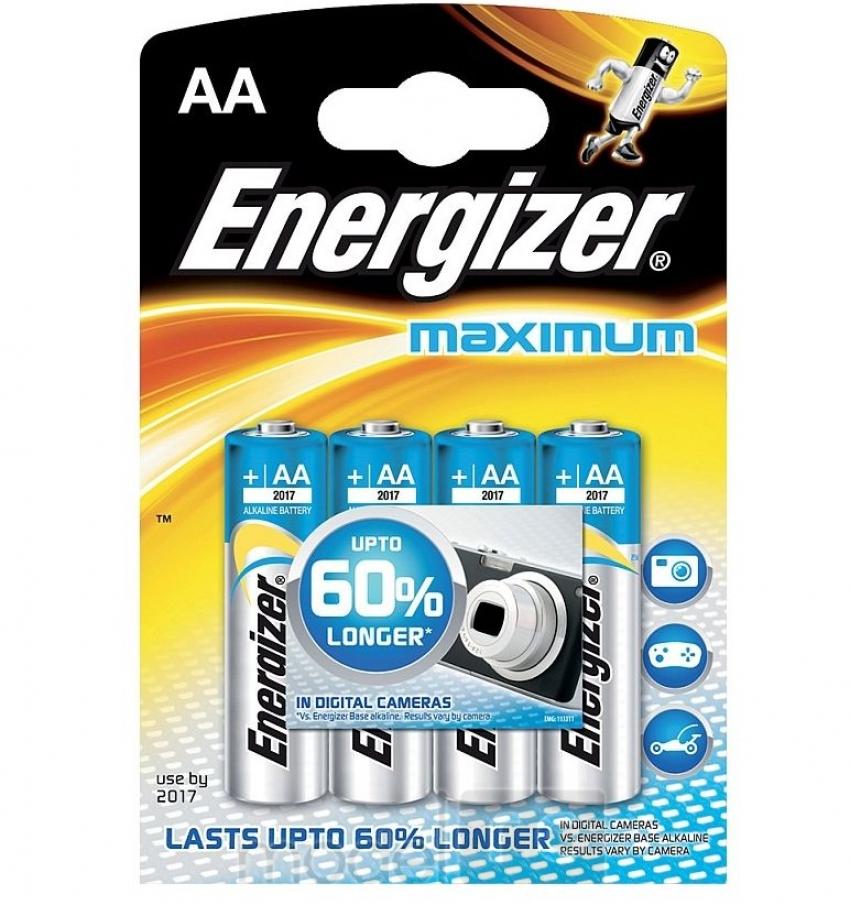The image features a rectangular package of Energizer AA batteries designed for retail display. The top of the package prominently displays the brand name "Energizer" in bold white letters. On the upper left-hand side, the text "AA" indicates that the package contains 1.5-volt AA batteries. 

On the right side of the package, there is a depiction of the iconic Energizer battery mascot, complete with arms and legs, appearing to run. Below the brand name "Energizer," the word "MAXIMUM" is printed in light blue letters.

The package contains a total of four batteries, clearly visible and arranged vertically. Each battery is detailed with a light blue top featuring a white plus sign, followed by the text "AA" in white letters. Directly beneath this, the year "2017" is printed in black.

A yellow swirl design encircles the background, complementing the overall visual aesthetic. At the bottom, the word "Energizer" appears again, this time in black font outlined in white.

The packaging itself is designed to be hung on a hook, with a circular hole at the top center. The upper part of the package is black, gradually transitioning to a neon yellow-orange gradient, enhancing its visibility on retail shelves.